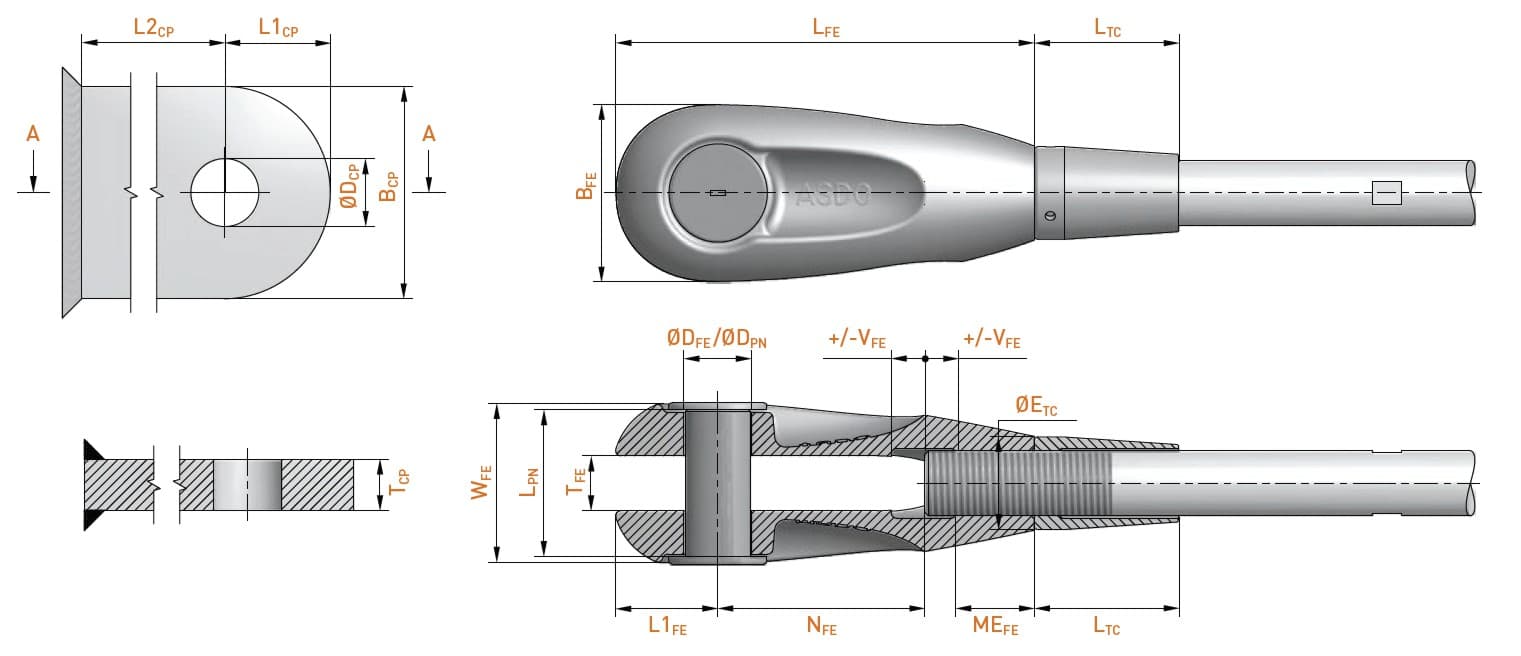The image presents a detailed technical drawing showcasing a metal object with a cylindrical and straight shape, likely resembling a tool such as a socket wrench or a gun-like mechanism. Highlighted from a top angle view, the blueprint meticulously details various sections with precise measurements and annotations such as LFE, LTC, and BFE. The drawing consists of four distinct views: an exterior side view, an interior side view, and two internal cross-sections. Gray on a white background, the annotations and dimensions are illustrated with golden-brown text and black measurement lines and arrows, detailing distances and circumferences essential to the design. The object features a button near the bottom, suggesting functionality requiring manual operation. Overall, it seems to be a comprehensive guide to the construction and dimensions of a technical instrument, possibly meant for patent purposes.